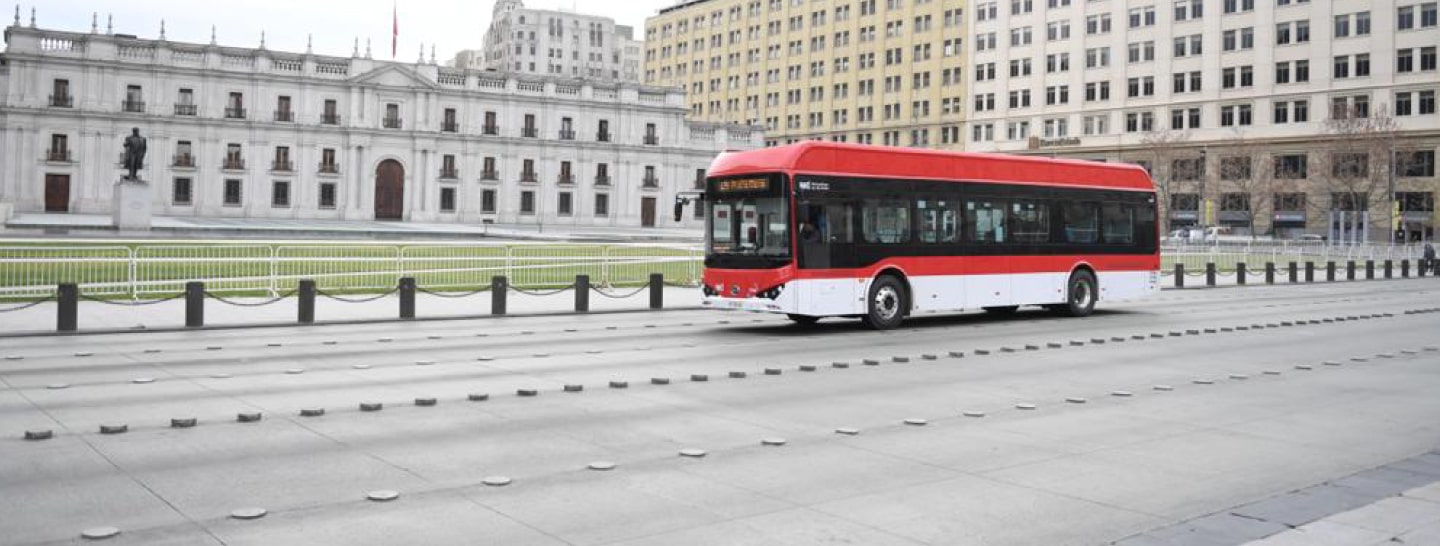The image depicts a red and white city bus parked on a multi-lane, concrete roadway in a bustling urban environment. The bus features a white strip along its bottom, extending across its two visible tires, and is labeled with yellow lettering on the top front, possibly indicating its destination. The bus is positioned next to a guardrail made of concrete or wooden poles strung together, while a white picket or steel fence runs parallel to it.

In the background, there are several noteworthy buildings. To the left, a three-story white building with a brown door can be seen, flanked by a tall, ten to twelve-story structure composed predominantly of windows, transitioning from tan to white as you move across it. Additionally, there is a large, two-toned beige building that might serve as a hotel or office complex. On the city's skyline, a significant gray building with an arched doorway, possibly governmental, features a flag on top and a statue in front of a block pedestal, enclosed by a fenced grassy area.

The sky is overcast with white clouds, and there is a leafless tree indicating it is likely fall. Unlike a typically busy street, this scene appears quiet, with no visible traffic except for the stationary bus. The road itself is characterized by raised circular objects separating the lanes, and some cars, though faint, can be spotted in front of the distant hotel-like building.